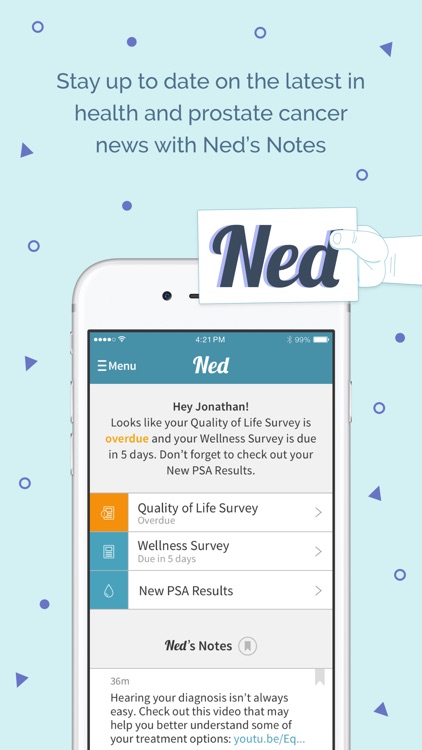This screenshot features a light blue background adorned with small, light blue circles rimmed with dark blue edges, interspersed with various dark blue circles and blue triangles. Prominently displayed at the top, the text reads, "Stay up to date on the latest in health and prostate cancer news with Ned's Notes."

Occupying the majority of the image, an animated phone with a white cover is the focal point, accompanied by an animated hand above it, holding a white sign that reads "Ned" in dark navy font. The phone screen showcases a detailed interface.

The blue status bar at the top indicates the time as 4:21. Below, a navigation menu is evident, with 'Ned' displayed in white in the center. The message following that, targeting a user named Jonathan, states: "Hey Jonathan, looks like your quality of life survey is overdue," with the word "overdue" highlighted in orange. It continues to inform him that his wellness survey is due in five days and reminds him to check out his new PSA results.

Three categories are listed, each within colored boxes and accompanied by icons and right-facing carets:
1. In an orange box: "Quality of Life Survey," marked as "overdue."
2. In a blue box: "Wellness Survey," due in five days.
3. In another blue box: "New PSA results."

Further down, a section labeled "Ned's Notes" shows that 36 minutes ago, a message was posted: "Hearing your diagnosis isn't always easy. Check out this video that may help you better understand some of your treatment options," followed by a truncated web address.

This detailed depiction captures the essence of the screenshot, highlighting its informative and user-friendly design.